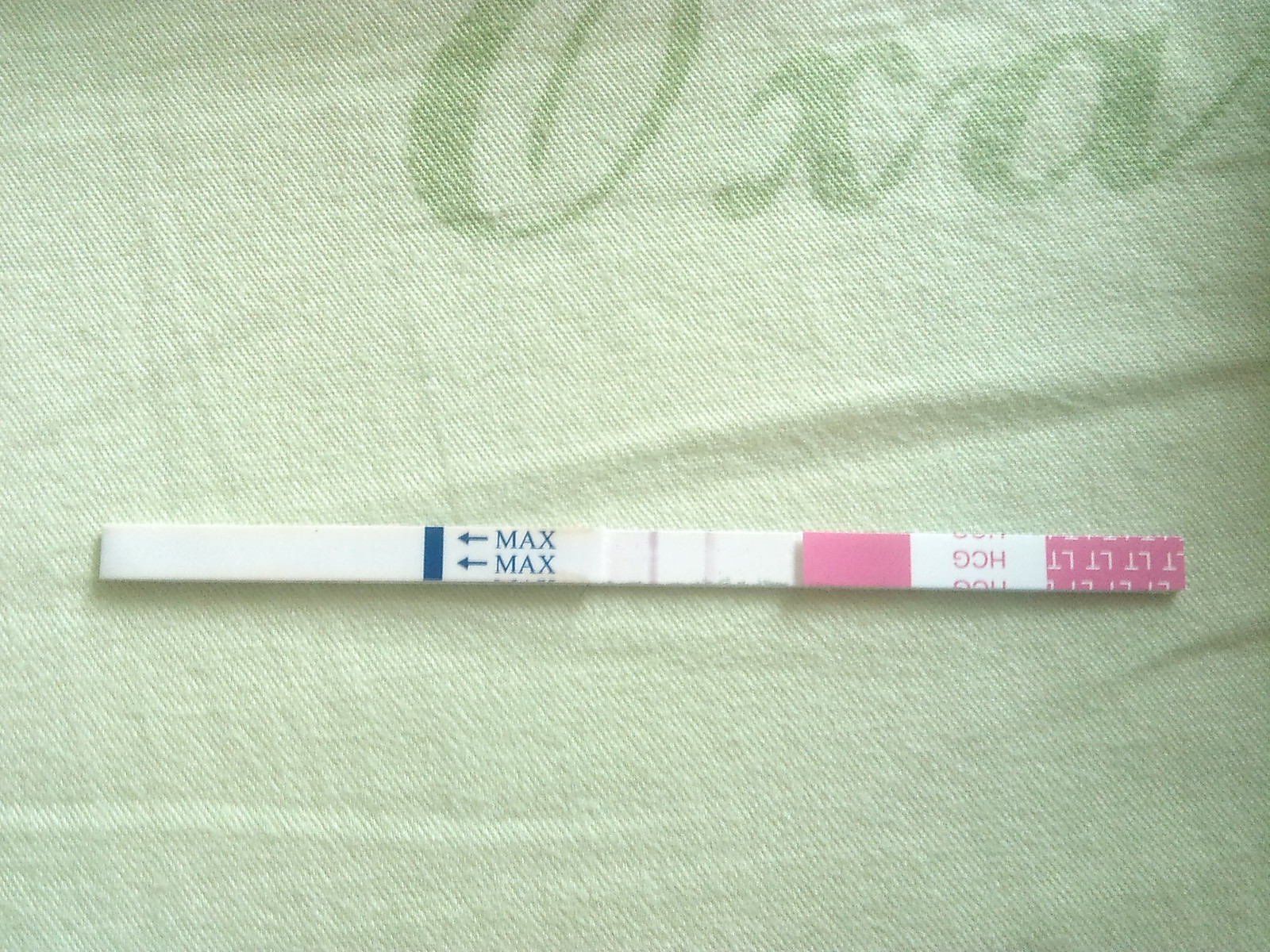The image depicts a piece of fabric, potentially greenish or gray, with distinctive features. Across the top, there are large, cursive letters "O," "X," and "A." At the center, a wide, long white strip runs horizontally, with additional white areas on both the left and right sides. Towards the far right, there's a pink section labeled "LT," and adjacent to it lies a white square containing pink letters, spelling "HCG." On the far left, there is a small pink square. The middle section features the word "MAXMAX" on the left-hand side and blue arrows pointing towards a blue strip. Below this, there is an elongated white rectangle. The fabric itself appears textured with some folds and is made up of stitched threads, giving it a slightly thick appearance. The image quality is low and grainy, with a slight shadow cast by a stick-like object across the fabric. In the central area, faint light blue stripes run vertically, adding to the composition's complexity.